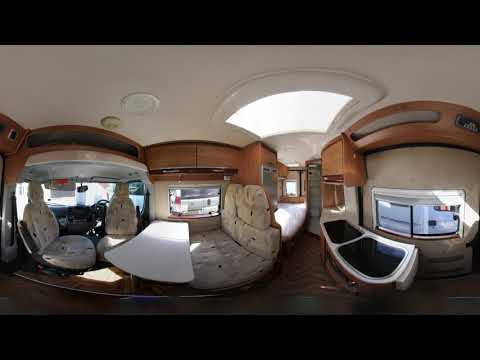The image is a 360-degree panoramic view of the inside of a motorhome, featuring a slightly distorted, circular appearance. The ceiling is white with a large, square skylight in the center, bordered by beige. On the left side of the image, there's a cozy seating area resembling a camper or van interior, with furry seats surrounding a table, and in the background, you can see the driver's area, including swivel chairs and a steering wheel. Towards the right side, there's a double sink or possibly two bathtubs, next to old-school brown wooden cabinetry. There’s also an induction cooktop near the door. Behind the chairs, there's a small bed, and possibly a refrigerator or a walkway leading to a small bathroom. The image additionally has top and bottom black horizontal bars framing the panorama, enhancing the overall distorted effect.